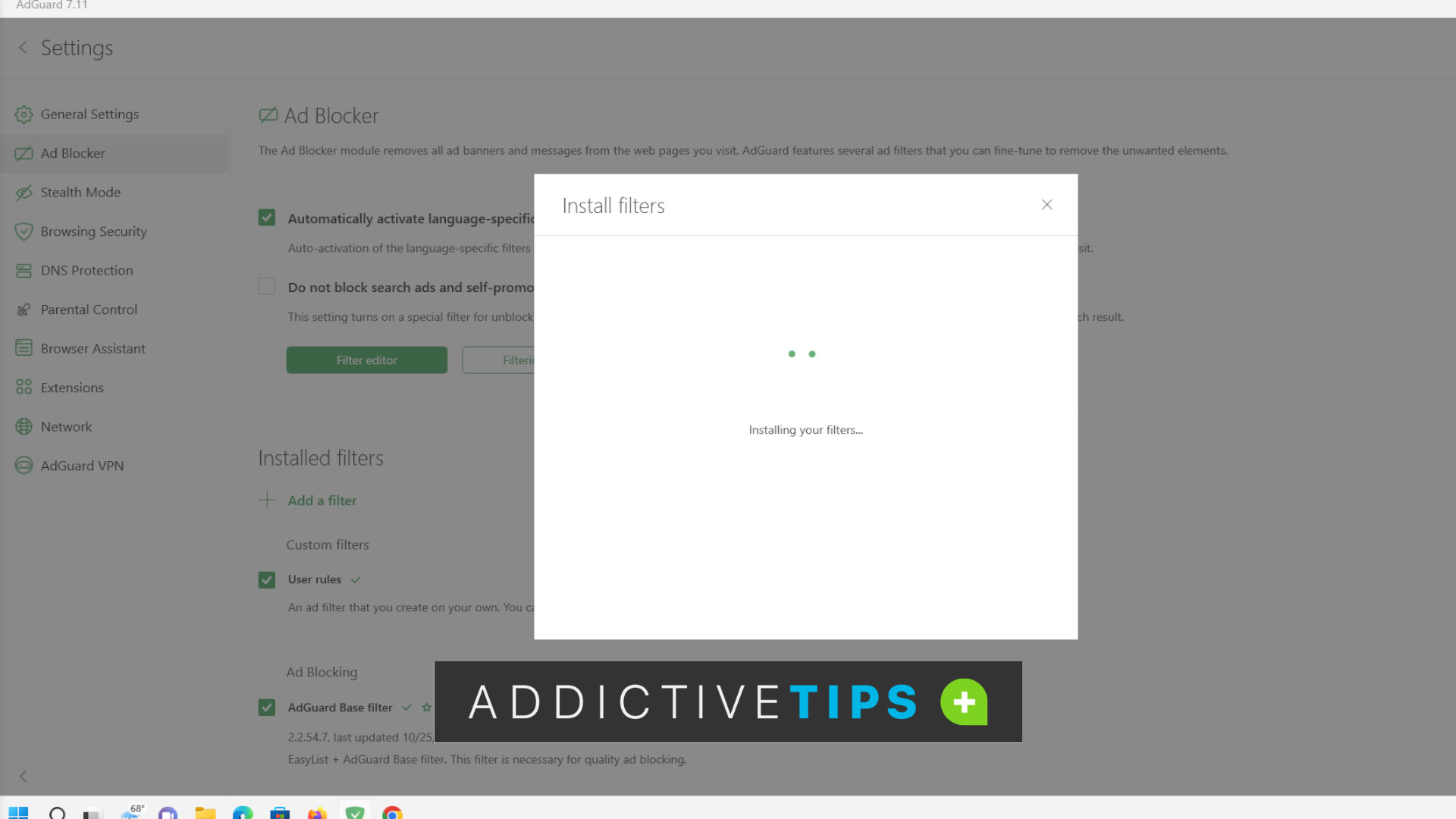This is a detailed screenshot of a website interface with a dark gray background. On the left side of the image, there is a vertical menu displaying a list of options: "General Settings," "Ad Blocker" (which is currently selected), "Stealth Mode," "Browsing Security," "DNS Protection," "Parental Control," "Browser Assistant," "Extensions," "Network," and "AdGuard VPN."

Dominating the center of the image is a white square with the heading "Install Filters" at the top. Inside the square, there are two green dots situated in the middle, followed by the text "Installing Your Filters." 

Below this white square is a prominent black banner. The banner features the text "ADDICTIVE TIPS" in all caps; "ADDICTIVE" is written in bold white letters, while "TIPS" is in bold blue letters. Adjacent to this text is a green teardrop shape with a white plus sign at its center.

At the very bottom edge of the image, there are partially visible computer icons, but they are cut off and not fully discernible. The overall dimensions of the image indicate that it is wider than it is tall. The screenshot is entirely illustrative, with no photographic elements present.